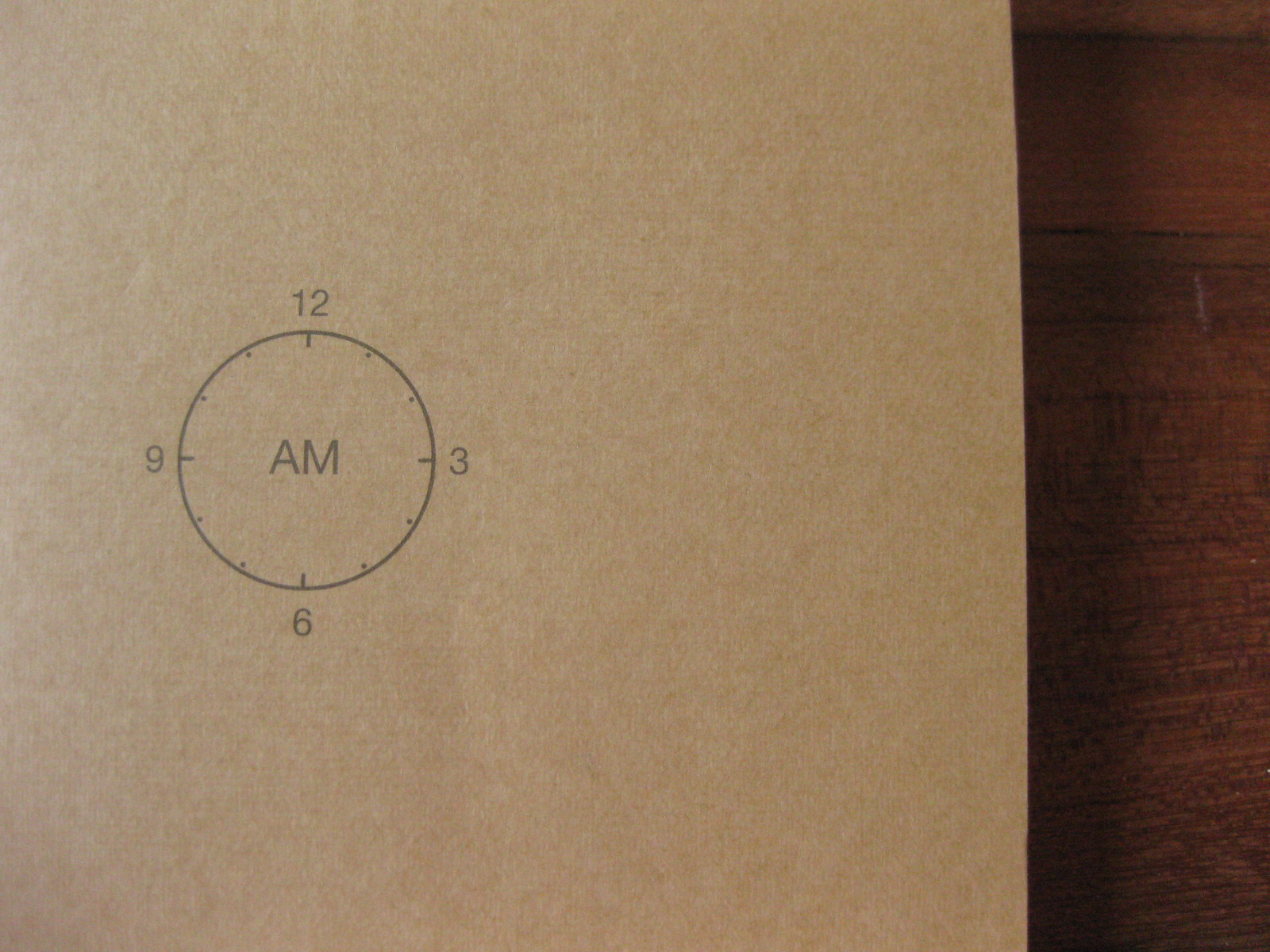This photograph captures a tan piece of paper resting on a cherry wood surface, with the intricate wood grain visible beneath. The paper features an embossed gray image of an abstract clock. The minimalist clock design prominently displays the numbers 9, 12, 3, and 6, each marked with thin lines, while small dots replace the other numbers around the clock’s face. The center of the clock showcases the word "AM" in a gray font. There are no other objects or images present in the photograph, drawing complete focus to the detailed and unique clock depiction.